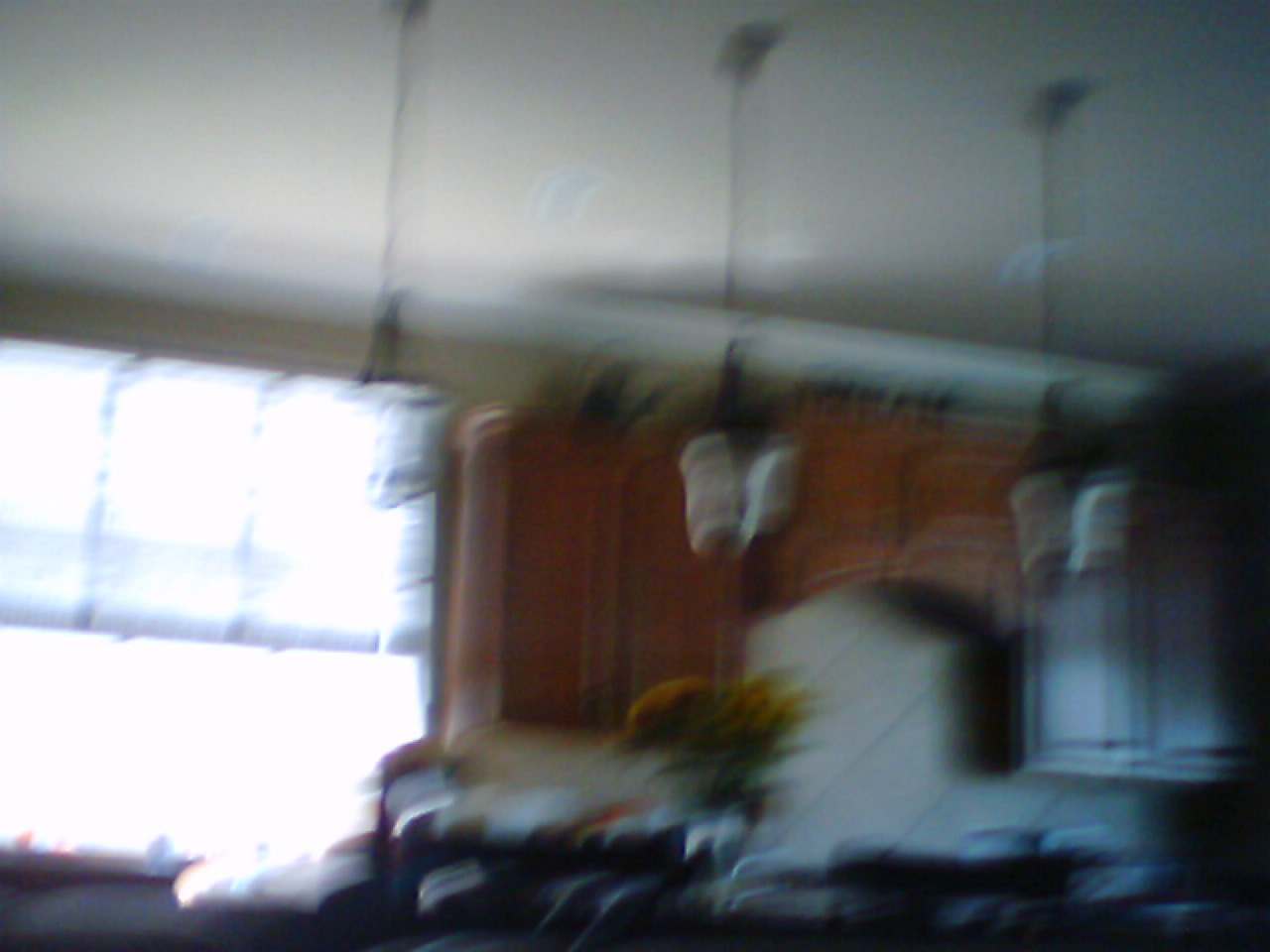This is a blurry photograph of a kitchen that captures a white ceiling from which three black cords hang, each suspending a white lamp that illuminates the surface below. The surface is cluttered with various items, adding to the lived-in feel of the space. In the background, there is a large window nearly reaching the ceiling, allowing bright sunlight to pour into the room. Wooden cabinets with a reddish-brown stain frame the scene, including vertical cabinets and arched ones that contribute to the kitchen's rustic charm. Dominating the center of the image is a table adorned with a vase of vibrant orangish-yellow flowers with lush green leaves, adding a pop of color to the setting.